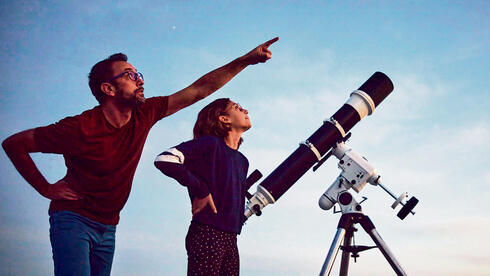This is a color photograph of a star-watching scene featuring two individuals and a large telescope. On the left, a man with short brown hair, glasses, and a beard and mustache is dressed in a red t-shirt and blue jeans. He stands with his right hand on his hip while pointing upwards to the upper right with his left hand. To his right, a woman with short brown hair and glasses, dressed in a blue top with white-striped sleeves and black pants with white dots, mirrors his stance, also resting her hand on her hip as she gazes towards the upper right. The large telescope, equipped with a black cylinder and white components, is mounted on a metal tripod and aligned in the same direction as the man’s gesture. The backdrop captures a twilight sky transitioning from blue to subtly pinkish-orange hues, indicating dusk, with a single star visible near the top of the image. The scene exudes a sense of shared wonder, as the pair appear to be preparing to map out celestial objects during a clear spring or summer evening. The intimate setup and clear focus on the telescope suggest a harmonious blend of casual stargazing and educational purpose, hinting that the man might be teaching the woman, possibly his daughter, about the stars.